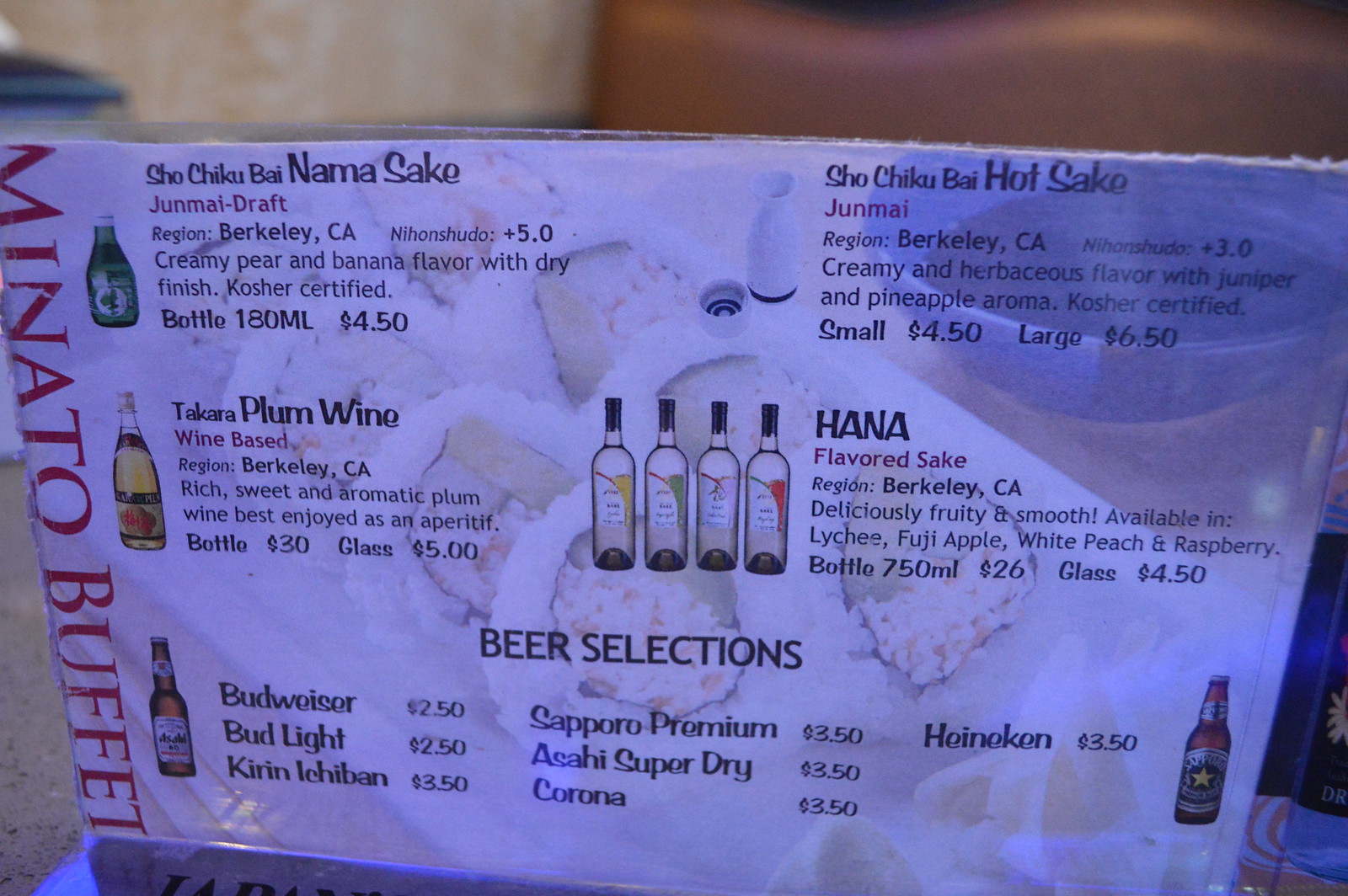The image depicts a drink menu from Minato Buffet in Berkeley, California, presented vertically in red on the left-hand side. The Shochiku by Namasaki Junmai Draft Sake, a kosher-certified beverage from Berkeley, offers creamy pear and banana flavors with a dry finish. It’s available in a 180 ml bottle for $4.50. The menu also lists Takara Plum Wine, a rich, sweet, and aromatic wine-based aperitif also from Berkeley, available for $30 a bottle or $5 a glass. Beer selections include Budweiser and Bud Light for $2.50 each, and several other options like Kirin Ichiban, Sapporo Premium, Asahi Super Dry, Corona, and Heineken, all priced at $3.50. Additionally, the menu features Shochiku by Hot Sake with a creamy, herbaceous flavor of juniper and pineapple aroma, available in small for $4.50 and large for $6.50. Hana flavored sake, known for its fruity and smooth profile, comes in lychee, Fuji apple, white peach, and raspberry varieties, priced at $26 a bottle or $4.50 a glass. The menu is set against a blurred restaurant counter background, with faint images of the drinks and food dishes.